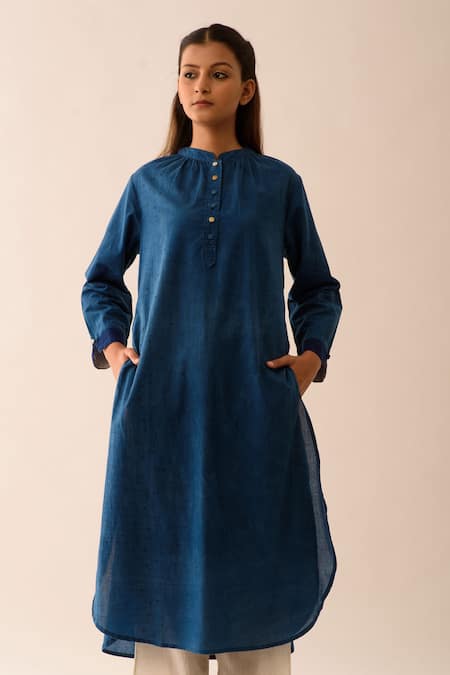This is a photograph of a young woman with long, dark hair parted in the middle, looking to her right against a beige background with a pinkish-gray undertone. She is wearing a long, loose-fitting blue tunic that reaches to her knees, with six buttons running down the front. The tunic features a high collar, two pockets at her sides where she casually rests her hands, with her thumbs sticking out. Beneath the tunic, she wears loose-fitting off-white pants. The woman has a subtle makeup look with red lipstick and mascara, and she is not wearing any jewelry. Her hair is parted in the middle, flowing naturally behind her ears and down her back.